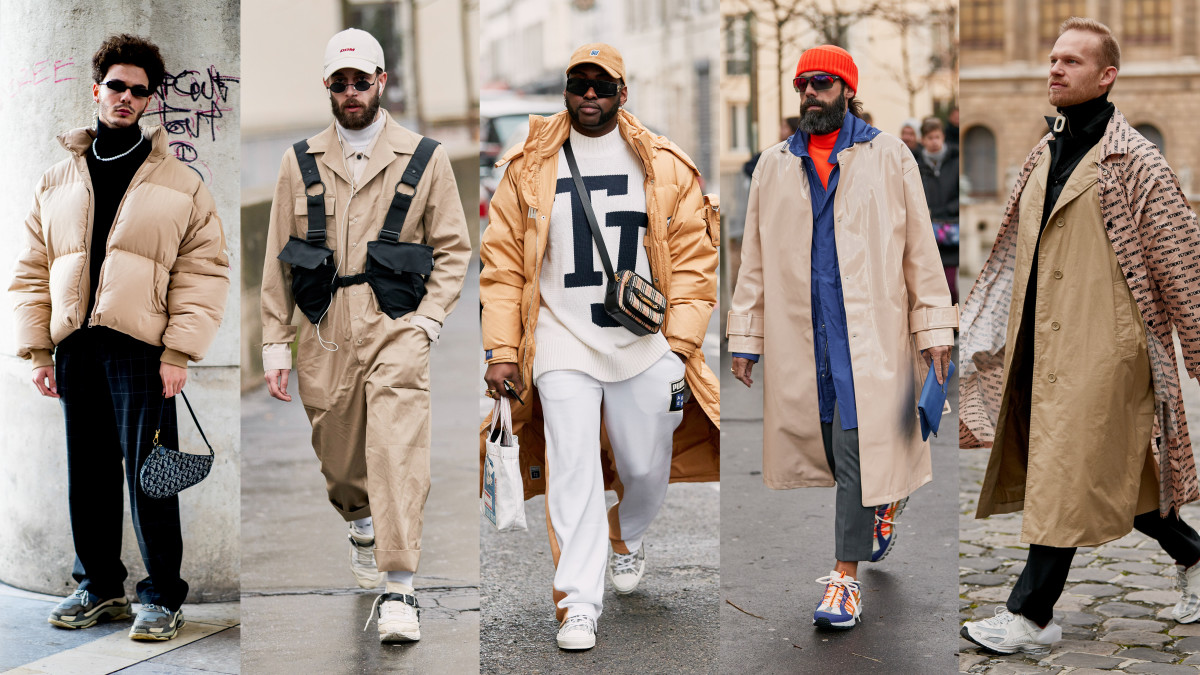This series of five separate photos captures a high-fashion urban ensemble, each featuring a different man against neutral, city-centric backgrounds. These images, clearly orchestrated for a fashion shoot, showcase the layering of diverse textures, patterns, and accessories, indicative of urban street style.

1. The first man stands confidently in front of a graffiti-adorned wall, donning a beige puffy jacket over a black turtleneck, accessorized with a silver necklace, and black pants. His look is completed with blue tennis shoes and black sunglasses. He holds a bum bag, contributing to the layered aesthetic.

2. The second frame portrays a man in motion, sporting a beige jumpsuit with a white baseball cap featuring red lettering. He carries two bags, a backpack and a crossbody, and complements his look with white sneakers that have black straps and ear pods, underscoring the contemporary urban style.

3. The third individual, also captured walking, wears a tan puffy jacket over a white Fendi sweater and white joggers with gold stripes. He accessorizes with a tan hat, sunglasses, and a white tote bag, suggesting a harmonious blend of function and fashion.

4. The fourth man is seen in a beige raincoat over a blue overcoat and an orange shirt, paired with shorter, gray pedal pusher pants. His orange hat matches his turtleneck, and he sports blue, white, and orange sneakers, along with sunglasses and a beard, embodying a bold yet coordinated streetwear look.

5. The final photo features a man sans sunglasses, wearing a black turtleneck layered under a textured shirt and a beige raincoat. His ensemble is rounded off with black pants, white sneakers, and another coat atop with indiscernible writing, highlighting the multi-layered trend within this fashion narrative.

Each man's distinct outfit contributes to an overall portrayal of high-fashion, urban elegance designed for a contemporary men's fashion magazine.